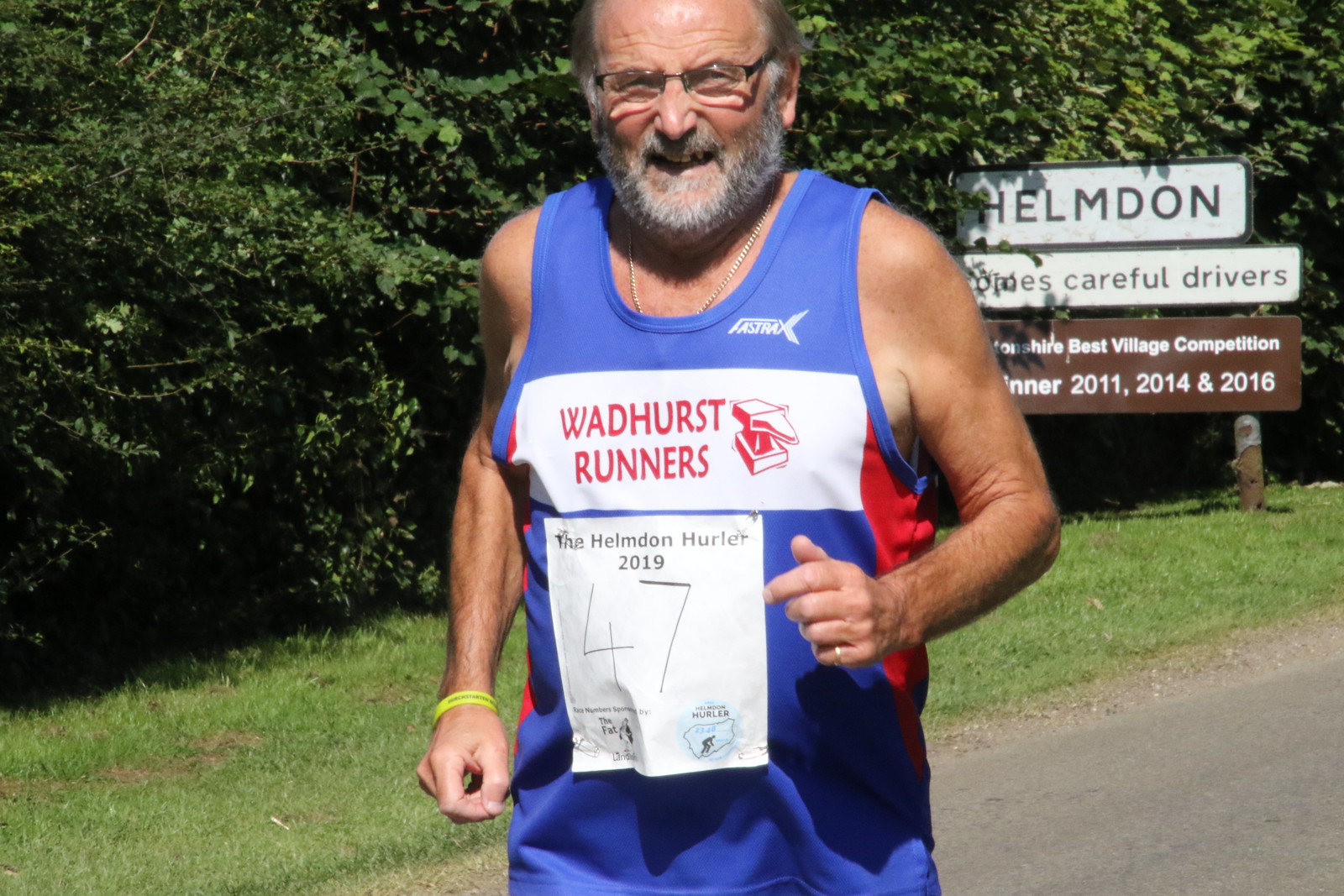In this full-color outdoor photograph taken on a bright, sunny day, an elderly gentleman is captured mid-run during a race. The man, positioned centrally in the image, sports a blue tank top featuring a white banner with red letters spelling "Wadhurst Runners" and an anvil graphic. Below this, a paper sign pinned to his chest reads "The Helmden Hurler 2019," with the handwritten race number 47. He has a short, scruffy gray beard, wears glasses, and is balding slightly. A gold wedding ring adorns his left hand, while a yellow wristband is visible on his right wrist. He also wears a chain around his neck. The man is running on a paved road bordered by neatly mowed grass, with a backdrop of dense, green trees. To the back right, a road sign reads "Helmden" with accompanying text about careful drivers and a blue sign underneath mentioning the "Shire Best Village Competition Winner 2011, 2014, and 2016."